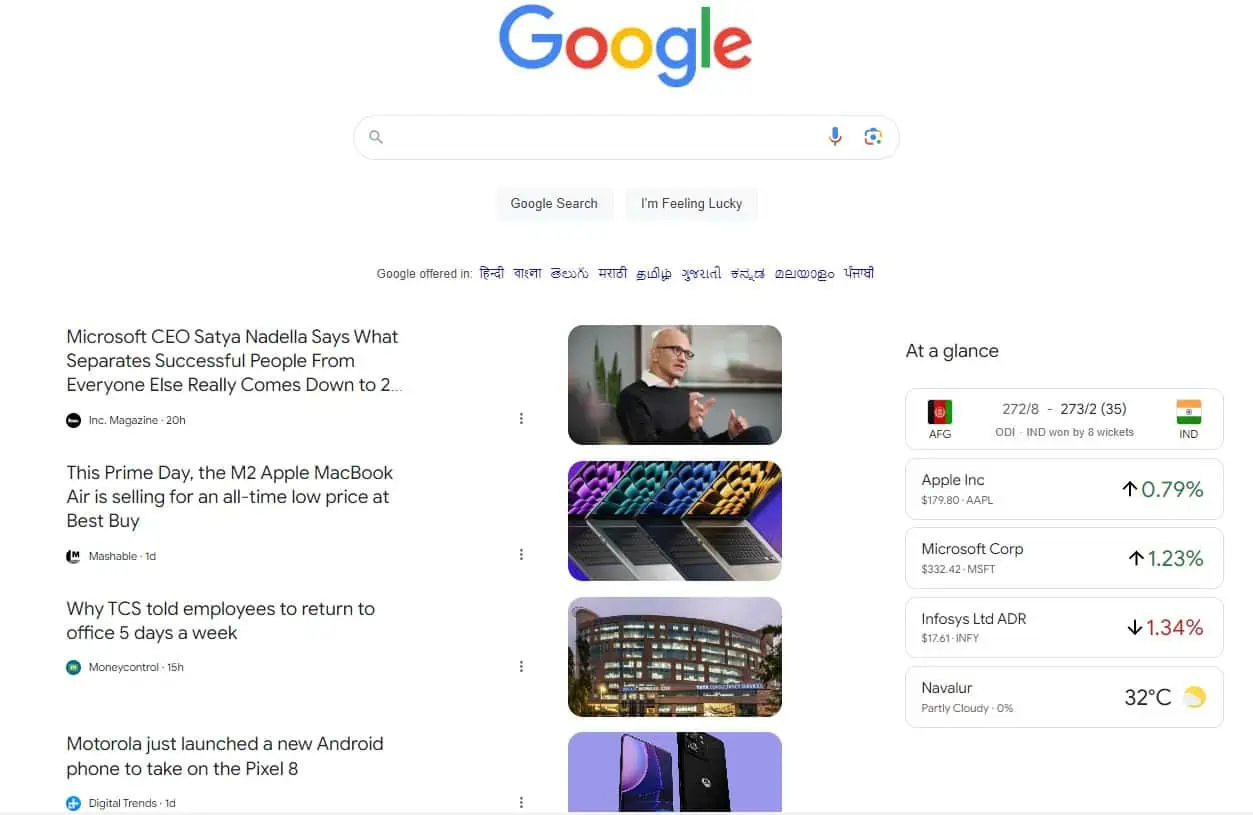Screenshot of Google Homepage Featuring Regional Language Options and At A Glance Updates

The screenshot captures the Google homepage, highlighting its interface for diverse users. The familiar Google logo and search bar dominate the page, inviting users to either "Google Search" or click on the "I'm Feeling Lucky" button for a random search experience. 

Just below the search bar, the page displays language options, specifically focusing on South Asian languages. Though not all scripts are identifiable, Telugu and Hindi are mentioned as notable inclusions, showcasing Google's accessibility features.

Adjacent to the search section is a snippet of current news articles. The latest updates include a headline involving Microsoft CEO Satya Nadella discussing the traits that differentiate successful people, although the article is truncated with "dot dot dot." Other news summaries indicate topics related to Apple and the Motorola Android phone.

On the right-hand corner, there's an "At A Glance" section displaying live updates and information. This includes a recent cricket match result where India defeated Afghanistan by eight wickets. Additionally, several stock updates are listed, featuring companies like Apple, Microsoft, and Infosys. The temperature in Navalur, India, is also shown, marked at 32 degrees Celsius, providing a quick weather update.